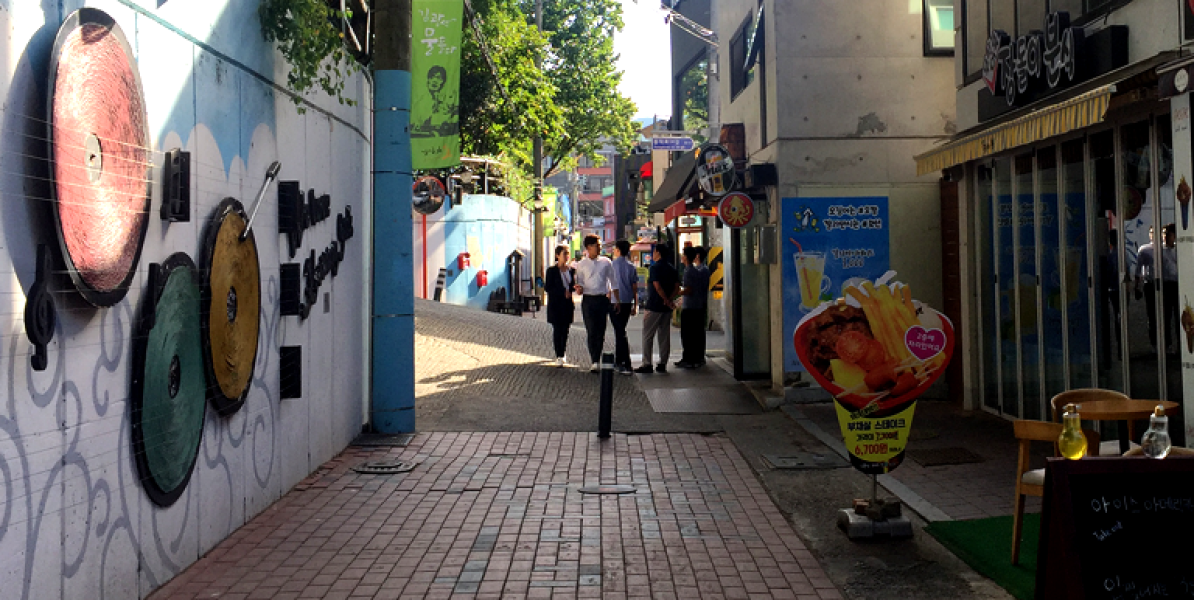A charming pedestrian street in a picturesque, likely non-U.S., location featuring a brick-paved thoroughfare lined with cafes and shops. One of the shops appears to serve fries and tomatoes among other offerings. The street is shaded and situated in a steep area, providing a break from vehicular traffic. Outdoor tables are set up along the street, adding to the leisurely atmosphere as several people stroll by. At one end of the walking street, there is an intriguing large wall adorned with giant circles and what seems to be remnants of an arrow or pipe embedded in it. The inclination of the adjoining streets emphasizes the convenience and safety of this dedicated pedestrian zone.